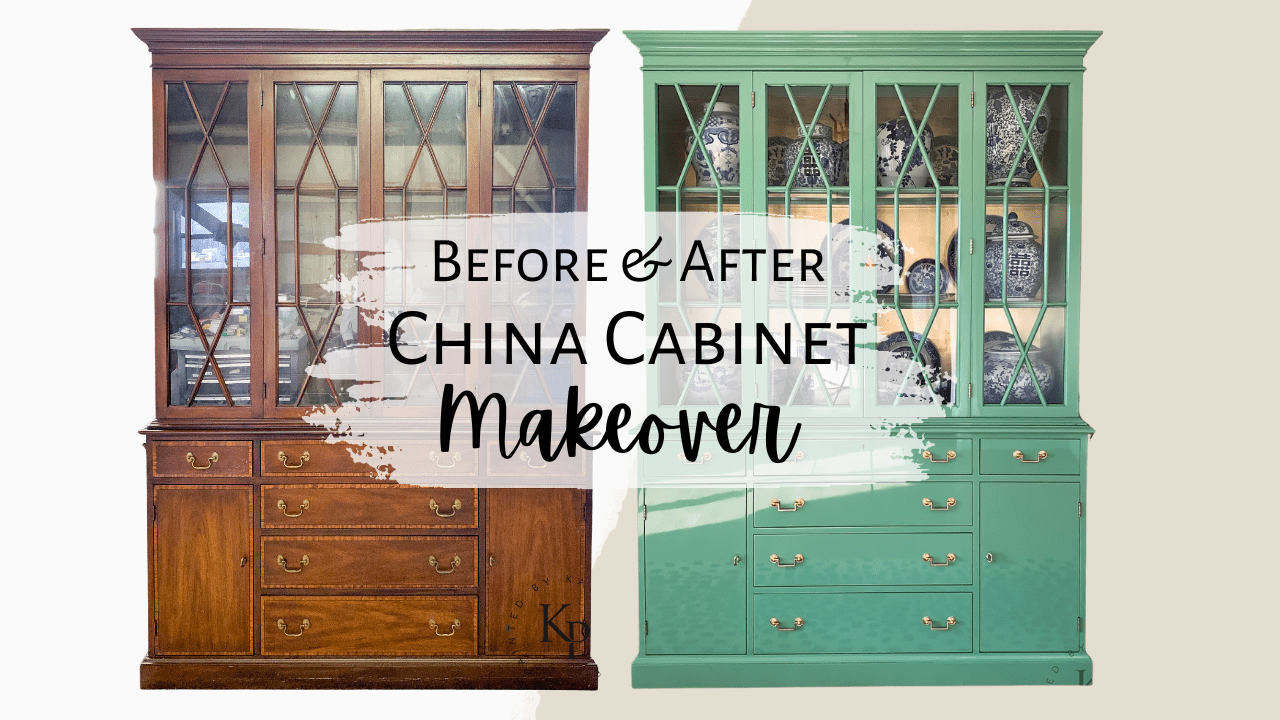This image showcases a before and after transformation of a china cabinet. The left side of the image presents the original cabinet in dark wood with four glass-paneled doors bordered by wooden strips in the hutch area. Below the hutch, there's a series of storage options: four central drawers, flanked by a smaller drawer each on the left and right, with bronze handles adorning the drawers and doors. The background behind the cabinet is nearly clear with a very dark tone. 

The right side reveals the cabinet post-makeover, now painted a light green with updated handles. The glass-paned sections display blue and white vases inside, adding a decorative touch. The background shifts to a tan color spanning from the top right to the bottom right corner. Centered across the image, in black letters against a white backdrop, is the text "Before and After China Cabinet Makeover,” with the word "makeover" elegantly scripted.